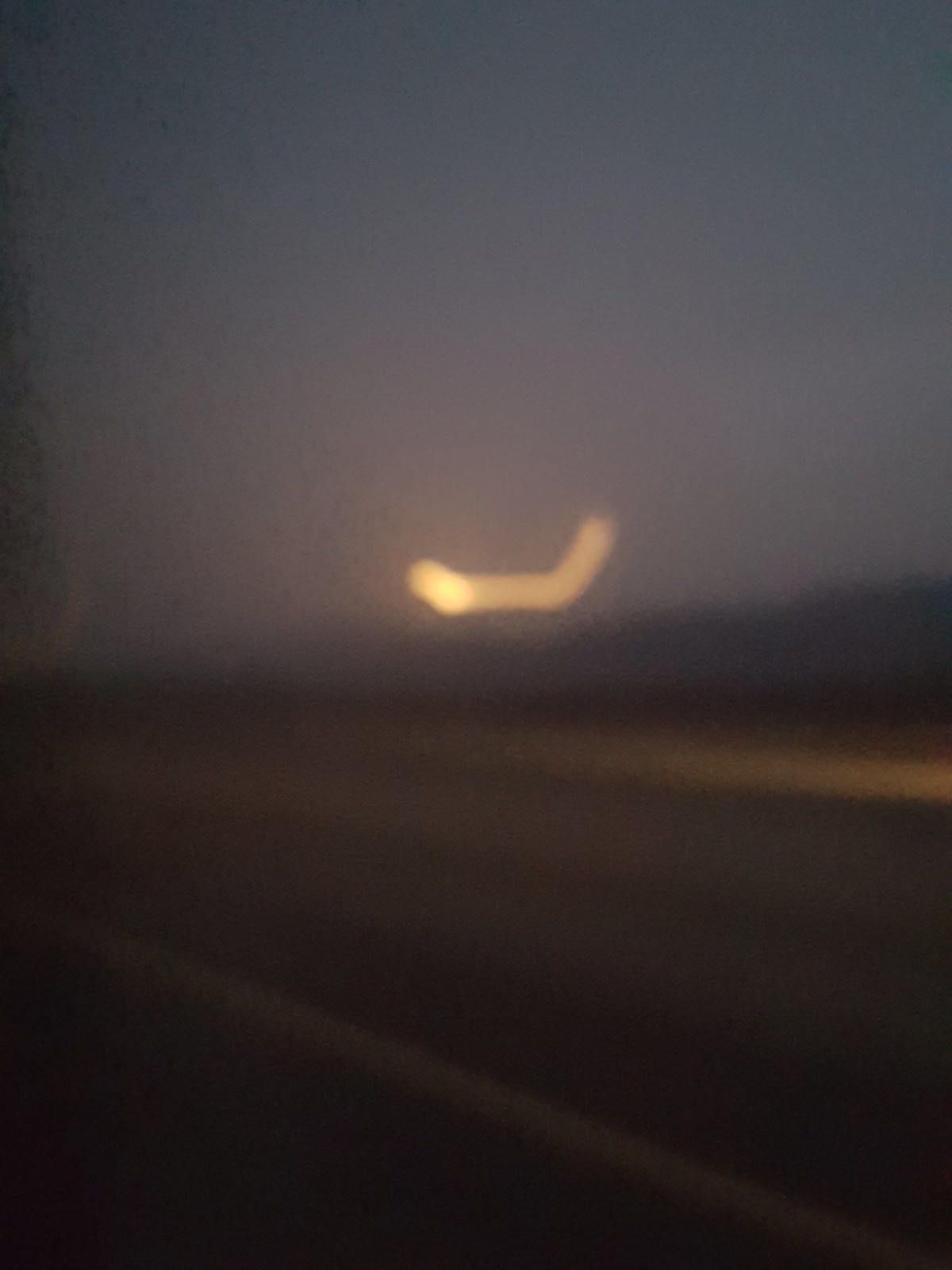This outdoor color photograph, although slightly blurry, captures a serene and somewhat eerie scene. An empty, single-lane highway devoid of any traffic stretches across the foreground. The road lacks a yellow dividing line, emphasizing its desolate and unused state. Behind the highway, a dense tree line creates a dark silhouette against the sky. The sky itself is dramatically dark, likely due to an eclipse in progress. A barely visible, crescent sliver of light—most probably the Sun—creates a striking focal point in the otherwise dim scene. This sliver emits a gradient of orange and pink hues that subtly illuminate the surrounding area. The overall mood of the photograph is quiet and somewhat mysterious, capturing the rare and captivating moment of an eclipse.